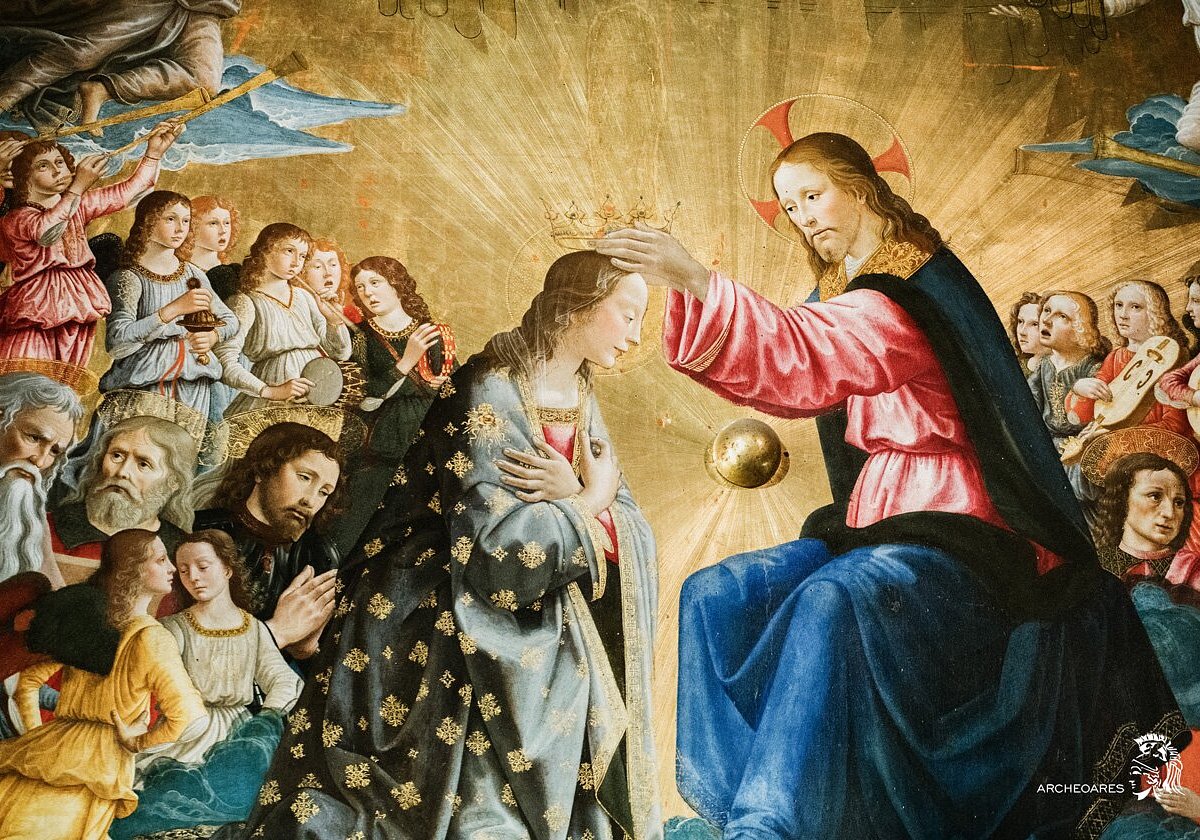This artwork is a detailed, medieval-style painting, set against a golden brown backdrop, depicting a significant Christian scene. At the center, Jesus is seated, clad in a pink loose-fitting shirt, a dark cape adorned with gold at the shoulders, and blue garment. He is identifiable by the halo around his head, symbolizing his holiness. Jesus is in the act of placing a crown on the head of the kneeling Virgin Mary, who has her arms crossed in reverence. Mary wears a shawl of black and light blue, and her long brown hair cascades down her back. 

Surrounding this central image are various figures, prominently men and women dressed in medieval attire. Some appear fascinated, watching the sacred event with awe. To the right of Jesus, amidst these spectators, is a figure playing a stringed musical instrument, reminiscent of a medieval lyre. Additionally, angels, both young and old, with bearded and mustached faces, are present, identifiable by their wings and angelic attire. Above Jesus and Mary, a floating golden orb can be seen, adding to the celestial ambiance of the scene. 

Near the bottom right corner of the painting is an inscription in white letters that reads "A-R-C-H-E-O-A-R-E-S," accompanied by a drawing that resembles a Roman centurion's profile. This painting, likely intended for a church or European museum, conveys a profound moment of divine coronation, celebrated by both heavenly angels and earthly witnesses.